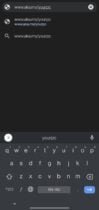A blurry screenshot of a smartphone browsing interface, showcasing a dark-themed webpage input screen. The background is black, contrasted with gray and white text. At the top, an address bar contains a partially visible URL, though it is too blurred to be deciphered. To the right of the address bar is a faint, blurry 'X' encased in a circle, likely for clearing the input. Below the address bar, there are two suggested URLs. At the very bottom of the screen, the dark gray predictive text or autofill bar is visible, accompanied by a dark gray keyboard with white letters.